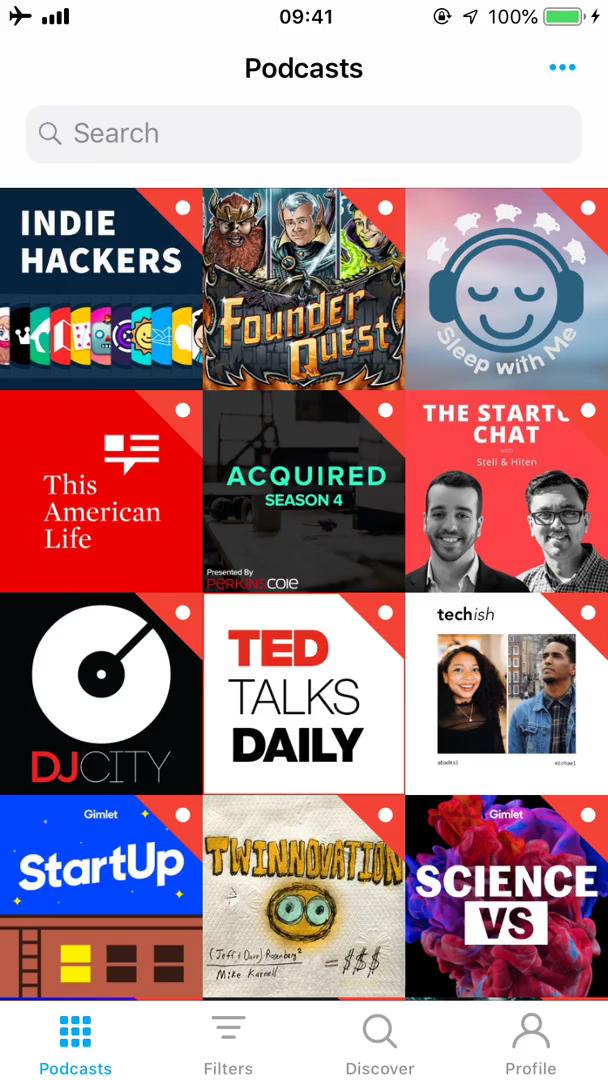This is a vertical screenshot of a smartphone's screen. Starting at the top left corner, there are several status icons - an airplane mode symbol, a Wi-Fi signal indicator, and the time displayed as 09:41 at the upper center. The top right corner features a directional arrow icon and the battery percentage, showing 100%, alongside a green battery icon.

Below the status bar, in the upper center, the word "Podcasts" is displayed in black. Directly beneath this is a gray search bar with a magnifying glass icon.

The main content area is a grid layout consisting of 12 rectangular podcast covers, arranged in 3 columns and 4 rows. Each cover features the podcast title and an associated image:
- Top left: "Indie Hackers"
- Top middle: "Found Request" with a video game-like graphic
- Top right: "Sleep with Me" displaying an emoji with headphones, closed eyes, and sheep circulating around its head
- Second row left: "This American Life" in a red square
- Below the second row left: "DJ City" with an image of a round white record
- Other podcast titles and images continue in a similar format down the grid

At the very bottom of the screen, below the podcast covers, there is a navigation bar with four icons:
- A blue podcast symbol
- Three more icons labeled Filters, Discover, and Profile

This screenshot provides a detailed overview of a podcast app interface on a smartphone.